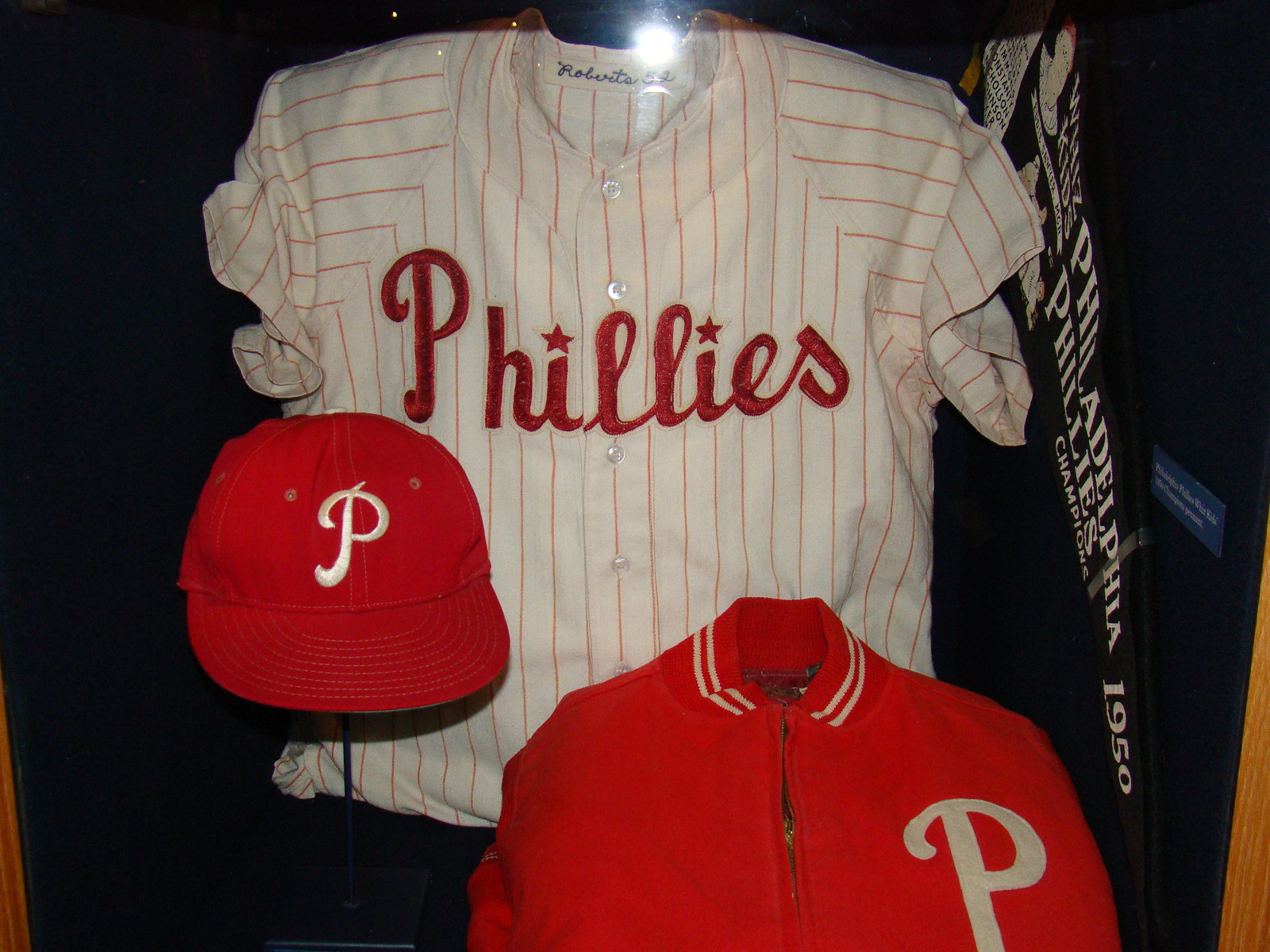The photograph captures an indoor museum display showcasing a vintage Philadelphia Phillies baseball uniform against a dark blue or black background. Central to the display is a white jersey adorned with vertical red pinstripes and short sleeves with horizontal red stripes. The front of the jersey features the word "Phillies" in red cursive letters, with stars dotting the 'i's. Accompanying the jersey is a red Phillies cap with a white "P" logo and a red varsity-style jacket with a letter "P" on the left breast, both stylishly propped up alongside the jersey. To the right of the display is a black triangular pennant that reads "Philadelphia Phillies Champions 1950." The entire ensemble is thoughtfully arranged with attention to detail, making it a nostalgic tribute to the baseball team's history. The composition is slightly marred by a camera flash reflecting off the glass panel of the display case.